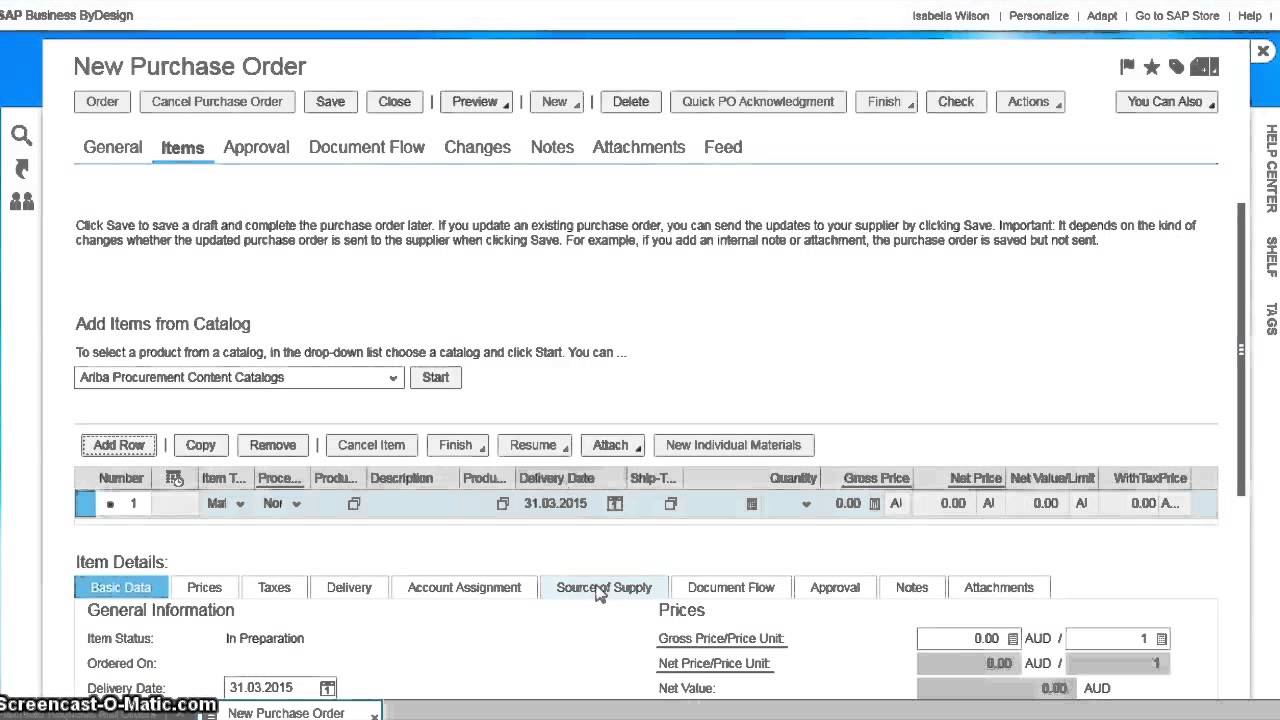The image depicts a webpage from the SAP Business ByDesign platform, specifically the interface for creating a new purchase order. The website features a predominantly white design. 

At the top of the page, the header includes various options such as "Isabella Wilson," "Personalize," "Adapt," "Go To," "SAP," "Share," and "Help." The title "New Purchase Order" is prominently displayed below the header.

The interface includes numerous actionable buttons: "Order," "Cancel Purchase Order," "Save," "Close," "Provide Now," "Delete," "Quick PO," "Acknowledgement," "Finish," "Check," and "Actions." On the right side of the page, a dedicated box presents some images which are not very clear.

The section headings "General" and "Items" are bolded and underlined with a teal line. Tabs such as "Approval," "Document Flow," "Changes," "Notes," "Attachments," and "Feed" are also visible. Below these tabs, there is a prompt instructing users to "Click Save to save a draft and complete the purchase order later. If you update an existing purchase order, you can send the updates to your supplier by clicking Save."

An important note highlights that the type of changes determines whether the updated purchase order is sent to the supplier upon clicking save. For instance, adding a referral note or an attachment will save the purchase order without sending it.

In the center, instructions direct users to add items from a catalog by first selecting a catalog from a drop-down menu and then clicking the "Start" button. The text within the drop-down is difficult to read but mentions something like "Albert Procurement Content."

Additionally, below this section are various clickable options for canceling, removing, or copying items, as well as viewing item details and the dollar amounts associated with the purchase order.